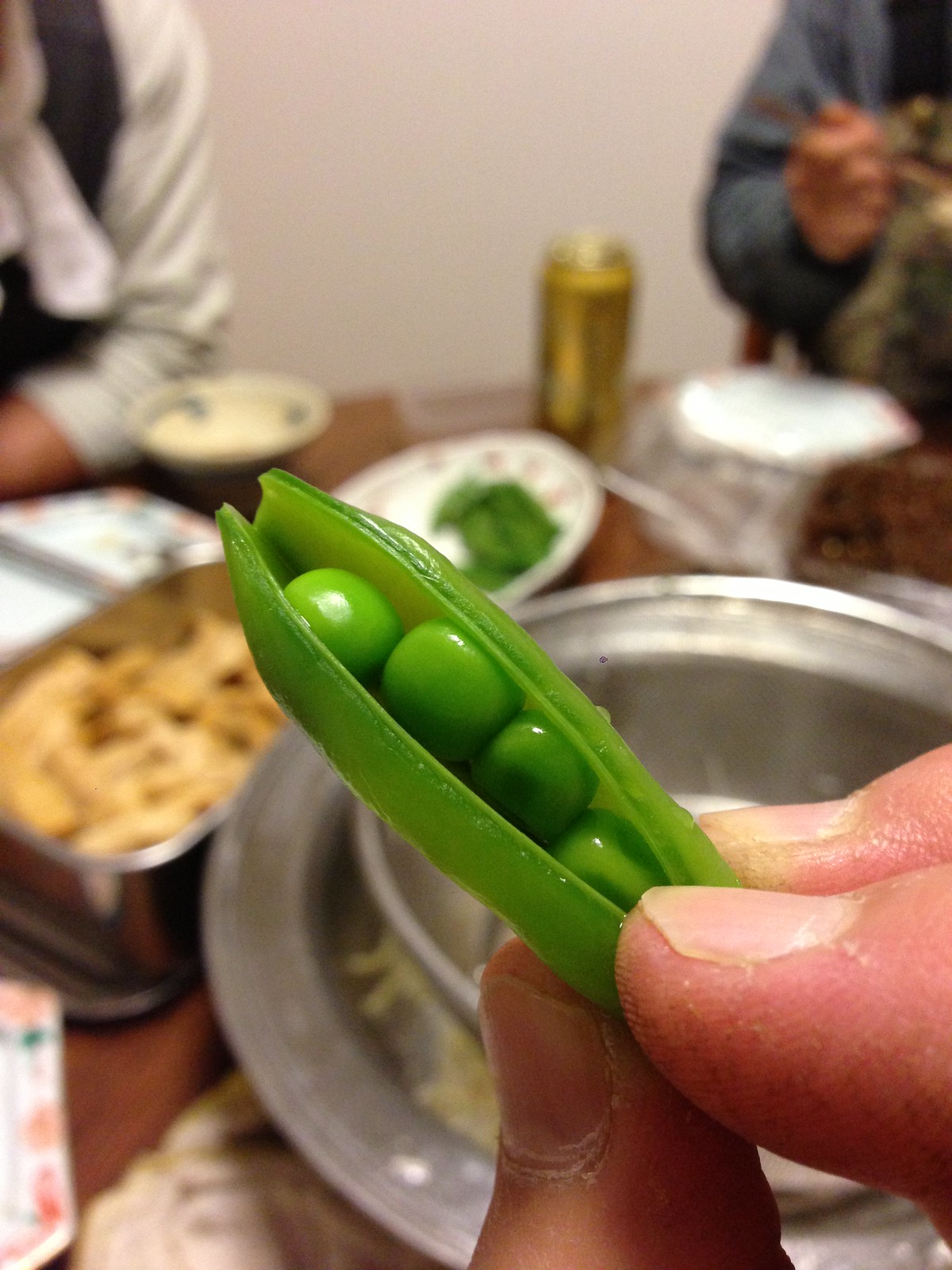The close-up image vividly captures a bright green pea pod held delicately by the fingers of a white person, prominently displayed in the right corner of the frame. The pod, which appears steamed and vibrant, is split open to reveal four shiny green peas nestled inside. Despite the sharp focus on the pea pod, the muted background reveals a bustling indoor dining scene with various elements vying for attention. A round silver bowl containing food accompanied by a serving spoon, a beige dish that possibly holds cauliflower, and a white plate with a hint of something green add layers of depth to the setting. Visible are also the blurred figures of a woman in a white long-sleeved shirt with a brown vest sitting beside a beige round bowl, and a man in a gray sweater, hand raised as if engaged in an activity, in front of a white plate and gold can. The scene, although fuzzy, conveys the warmth and activity of a shared meal.